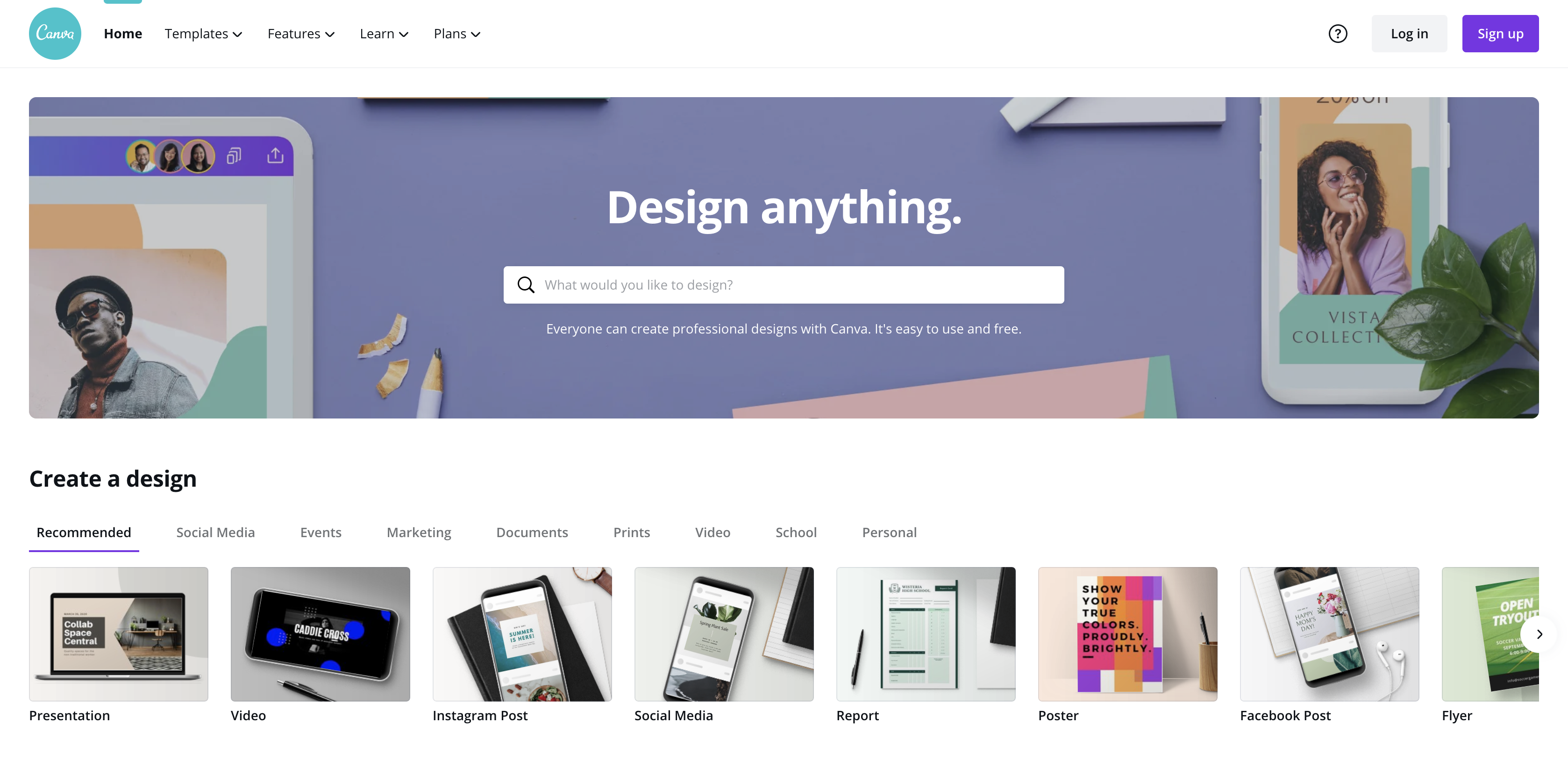The screenshot captures the homepage of the Canva web page, set against a white background. In the top left-hand corner, a blue circle with "Canva" written in white cursive script is prominently displayed. To the right of the logo, the navigation options "Home," "Templates," "Features," "Learn," and "Plans" are aligned horizontally, with a thin blue line above "Home."

In the top right-hand corner, there is a gray button labeled "Log In" next to a purple button that says "Sign Up." Beneath the navigation bar, a vibrant purple banner stretches across the width of the page. On the left side of this banner, a partial view of a white laptop screen shows a design in progress. The design features an image of a man wearing a burgundy shirt layered with a gray shirt and glasses. Adjacent to this, a white mobile device showcases an image of a woman wearing glasses, set against an orange background with green leaves visible on a table.

Centralized within the purple banner, in bold white text, reads "Design Anything." Directly below, a white search bar invites users with the prompt "What Would You Like to Design." Beneath the search bar, additional white text proclaims, "Everyone Can Create Professional Designs with Canva, it's easy to use and free." At the bottom of the banner, a call-to-action button states "Create a Design," accompanied by a range of options including "Presentation," "Video," "Instagram Post," and "Social Media," among others.